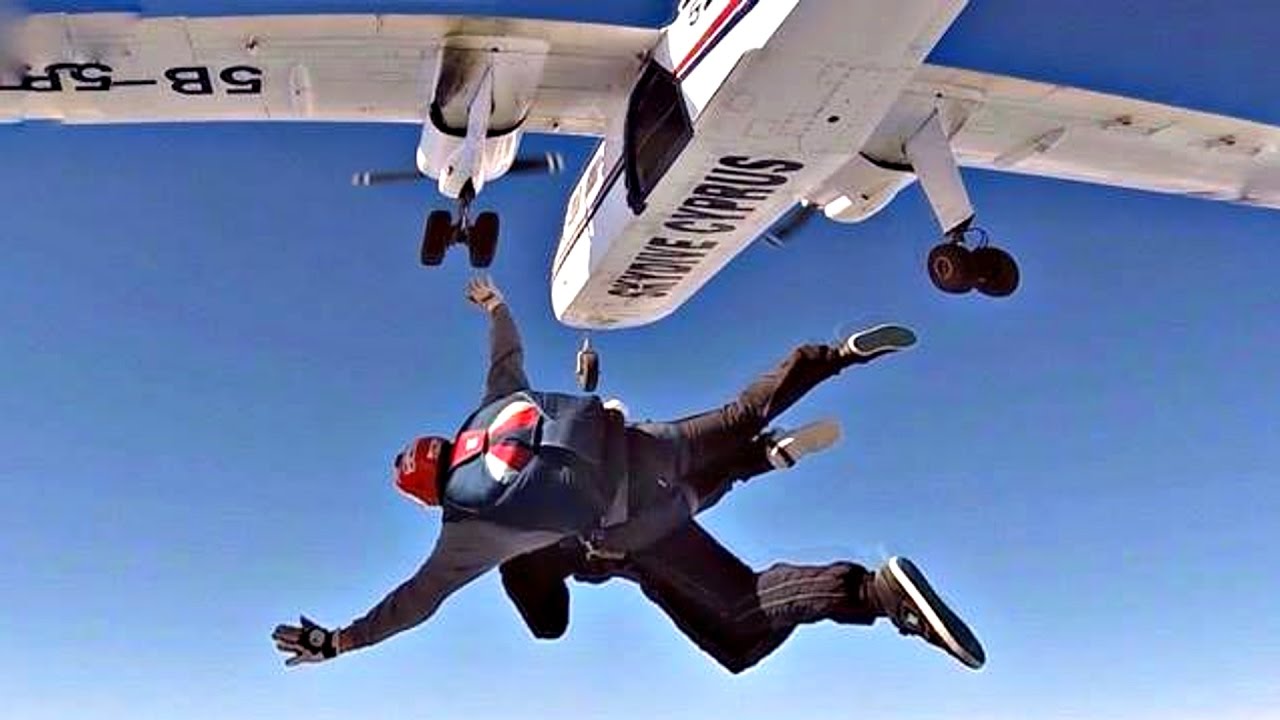In this vivid photograph, we capture the exhilarating moment of two people tandem skydiving after just leaping from a small, white airplane with its landing gear still out. The plane, utilized for skydiving as indicated by the blue "skydive Cyprus" lettering underneath, bears the markings "5B-5P" on the left side of the wing and there's a red and dark blue stripe along its side. In freefall beneath the clear, gradient blue sky, the skydiving duo is harnessed together, with the instructor at the back wearing a striking red helmet, grey gloves, and a blue, red, and white backpack parachute. The instructor's attire includes a dark long-sleeved shirt, black pants, and black sneakers with white stripes. Their arms are fully stretched out, embracing the fall, while the tandem skydiver seems less visible but also wears black attire. The contrast against the serene sky enhances the thrilling urgency of the jump, immortalizing this adrenaline-filled adventure.